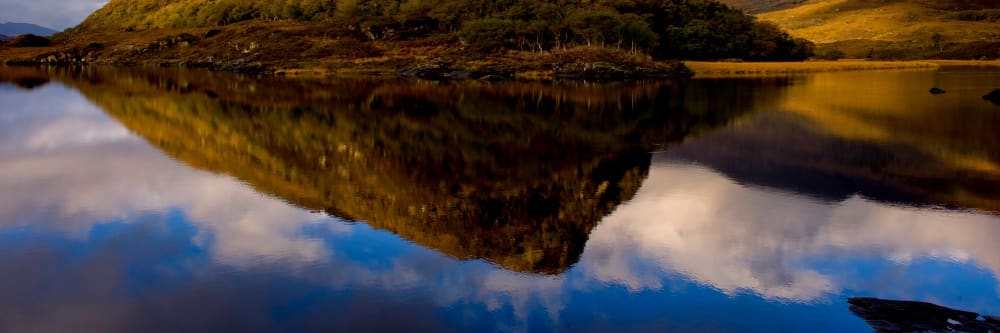The photograph captures a stunning landscape scene, potentially from the Highlands in Scotland or Ireland, showcasing a serene lake mirroring a vibrant blue sky filled with bright, puffy white clouds. The central focus is the reflection, which also captures a mountain range. This mountain has an intriguing blend of colors: dark brown with patches of yellowish-green, somewhat resembling the color of mold. Above the horizon, the real mountain and a small landmass, both with warm, rich green and yellow ochre hues, merge into the scene. The skies are a deep blue with both full and wispy gray clouds adding depth to the photograph. On the bottom right, a small landmass juts into the picture, contributing to the composition's dynamic balance. The overall image is rich with natural beauty and contrasting colors, offering a picturesque and tranquil view.